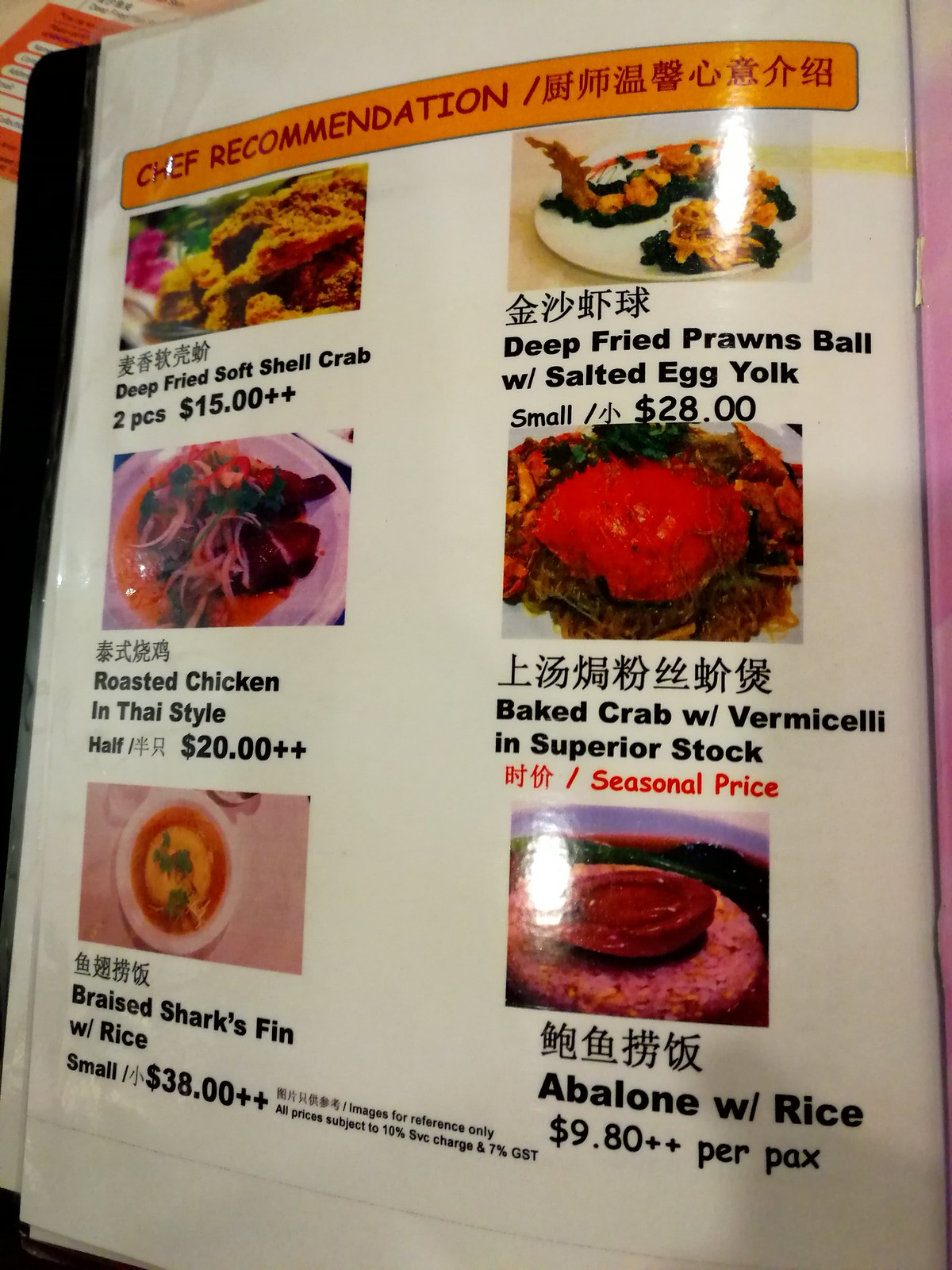The image depicts a menu from a Chinese restaurant, presented in a binder with clear plastic sheet protectors, allowing for easy updates to pages and prices. The binder itself appears to be black. The menu page shown is titled "Chef's Recommendation" and includes corresponding Chinese characters.

In the top left corner, there is an entry for "Deep Fried Soft Shell Crab" (two pieces) priced at $15, marked with two plus signs, and accompanied by a corresponding image of the dish.

Below this, there is a photograph of "Roasted Chicken in Thai Style," offered in half portion for half the price, and full portion for $20, again followed by two plus signs.

The subsequent item shown is "Braised Shark's Fin with Rice," with a small portion listed at $38 plus plus. Below this line, a couple of explanatory lines are present but not clearly visible.

In the top left corner of the menu, there is another entry labeled "Deep Fried Prawns Ball with Salted Egg Yolk," priced at $28 and accompanied by a photo.

Further down, another dish is listed as "Baked Crab with Vermicelli in Superior Stock" with a note indicating that the price is seasonal.

The final item displayed is "Abalone with Rice," priced at $9.80 plus plus per pack.

The detailed imagery of the dishes alongside the descriptive labels and specific pricing offers a comprehensive look at the restaurant's featured dishes.